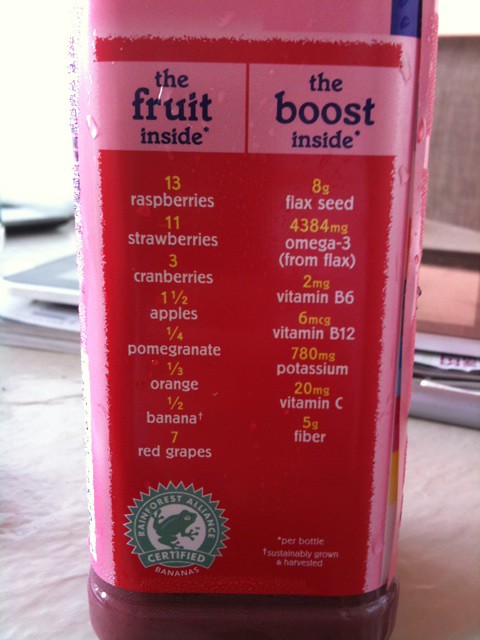This image captures a close-up shot of a square-shaped individual drink container positioned on a desk scattered with papers and folders in the background. The drink container features a vivid red label set against a contrasting pink background, adorned with a significant amount of text detailing its ingredients and nutritional information.

At the top of the label, a pink rectangular banner announces the fruit contents, listing, in descending order, "13 raspberries, 11 strawberries, 3 cranberries, one and a half apples, a quarter of a pomegranate, a third of an orange, half of a banana, and several red grapes." The ingredients are presented in white text with the respective quantities highlighted in yellow.

On the right, another section of the label is dedicated to the additional nutritional contents, stating "8 grams of flaxseed, 4,384 milligrams of omega-3 from flax, 2 milligrams of vitamin B6, 6 micrograms of vitamin B12, 780 milligrams of potassium, 20 milligrams of vitamin C, and 5 grams of fiber." The phrases "per bottle" and "sustainably grown and harvested" are mentioned at the bottom in smaller text.

Additionally, a teal-colored, sunburst-shaped seal is located on the right side of the label, featuring a white background in its center with a depiction of a frog. This seal signifies "Rainforest Alliance Certified," particularly emphasizing that the bananas used in the drink are sustainably sourced.